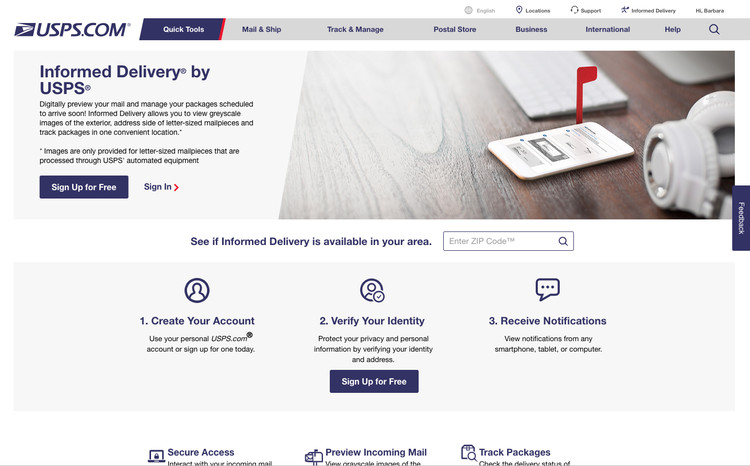The image appears to be a detailed informational page from USPS.com, possibly their homepage, but it’s not entirely clear. At the top of the page, set against a dark blue background, there’s a navigation bar with the following labels spread from left to right: USPS.com, Quick Tools, Mail & Ship, Track & Manage, Postal Store, Business, International, and Help.

Beneath this is a secondary navigation bar containing a visual icon on the left and the text "Informed Delivery by USPS." The description explains that this service allows users to digitally preview their mail and manage incoming packages. Specifically, it mentions that users can view grayscale images of the exterior address side of letter-size mail pieces and track packages all in one convenient location. Importantly, it notes that these images are only provided for letter-sized mail processed through USPS automated equipment. An invitation to "Sign Up for Free" is displayed in a dark blue box with white text, alongside a "Sign In" option in blue text with an arrow pointing right.

On the right side of the page, there's an image showing a cell phone on a desk. The phone has a red notification badge resembling the traditional flag on a physical mailbox, signifying incoming mail. The phone and notification are placed on a brown tabletop, partially showing the edge of a keyboard.

Below the primary description, additional informational content is provided to guide users in determining if Informed Delivery is available in their area. There’s a box where users can enter their zip code for this purpose.

The page also guides users through the setup process in three steps, presented on a light blue background:
1. **Create Your Account**: Use your personal USPS.com account to sign up. 
2. **Verify Your Identity**: Protect your privacy and personal information by verifying your identity and address.
3. **Receive Notifications**: View notifications from any smartphone, tablet, or computer.

At the very bottom, aligned right to left, are the labels "Secure Access," "Preview Incoming Mail," and "Track Packages." There is an additional line of text under these labels, but it’s partially obscured and unreadable.